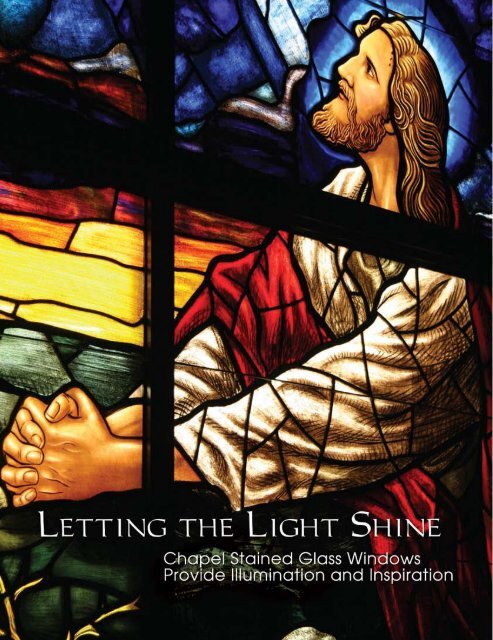The photograph showcases a beautifully detailed stained-glass panel depicting Jesus in a serene and prayerful pose. Jesus, with his long light brown hair and beard, is dressed in a white robe complemented by a red fabric draped over his arm. His hands, clasped together reverently, rest on a large rock before him as he gazes upward toward the heavens. The background is a vibrant display of stained glass in several colors, including yellows, reds, greens, and a particularly striking blue forming a halo around His head. At the bottom of the image, text in white letters declares, "LETTING THE LIGHT SHINE," followed by the subtitle, "Chapel stained glass windows provide illumination and inspiration." The intricate mosaic-style artwork is typical of what might adorn the side of a chapel, reflecting both artistry and spiritual symbolism.